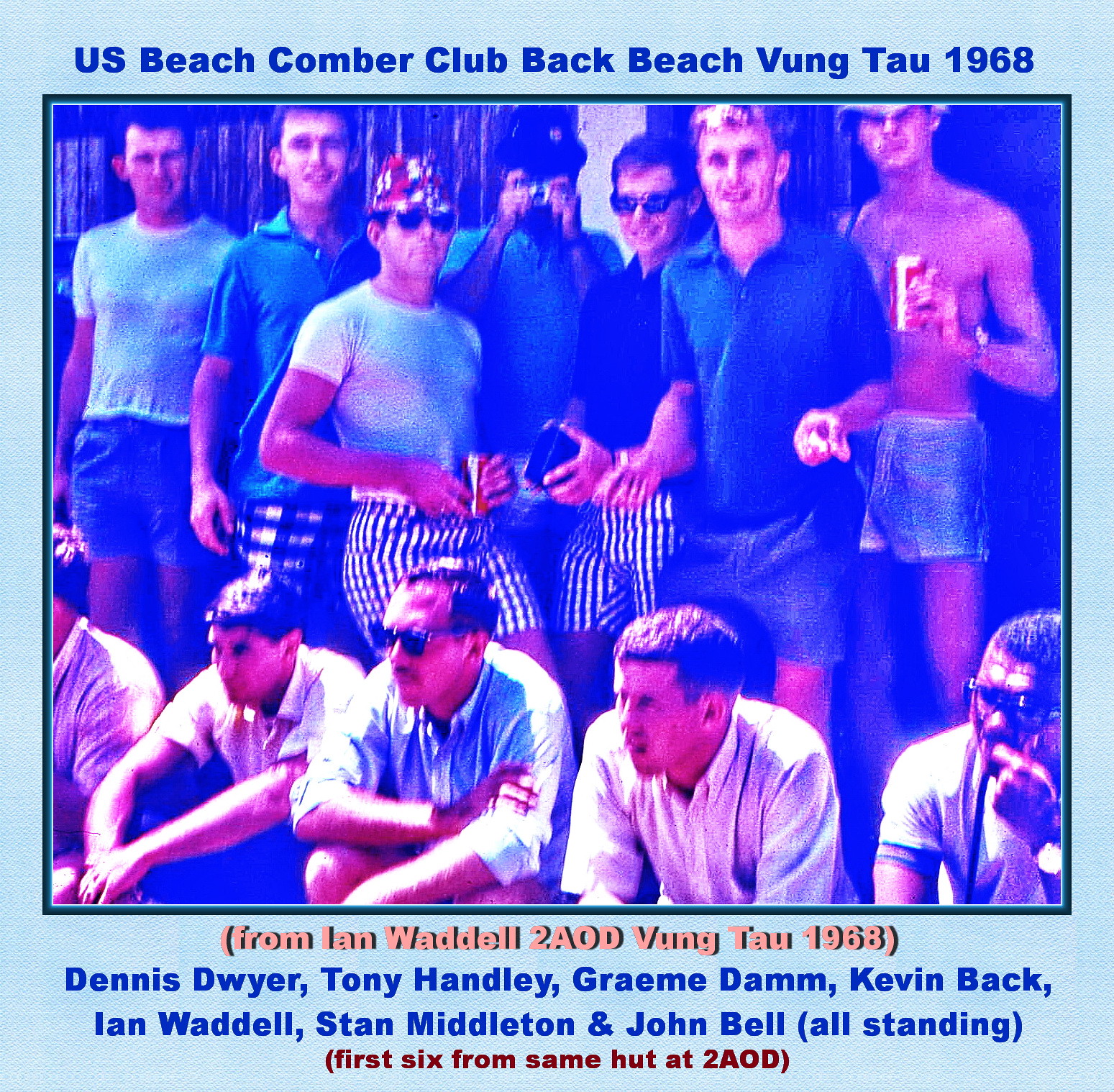This detailed image, dating back to 1968, depicts members of the U.S. Beachcomber Club at Back Beach, Vung Tau during the Vietnam War. Framed in a soft, eggshell blue border, the photograph itself carries royal blue hues. The top of the image bears a dark blue header reading, "U.S. Beachcomber Club, Back Beach, Vung Tau, 1968." Below the image in salmon-colored text is credited to Ian Waddell, "From Ian Waddell, 2A0, Vung Tau, 1968." The names of the men—Dennis Dwyer, Tony Hansley, Graham Dam, Kevin Back, Ian Waddell, Stan Middleton, and John Bell—are listed in blue over two lines, with a notation in red stating, "First 6 from same hut at 2A0D." The photo shows these young Caucasian men, standing casually, some sporting sunglasses and holding beverages, embodying a fraternity-like camaraderie. The entire setup, including landscape orientation, blends realism with graphic design elements, indicating a sense of nostalgia and reunion.